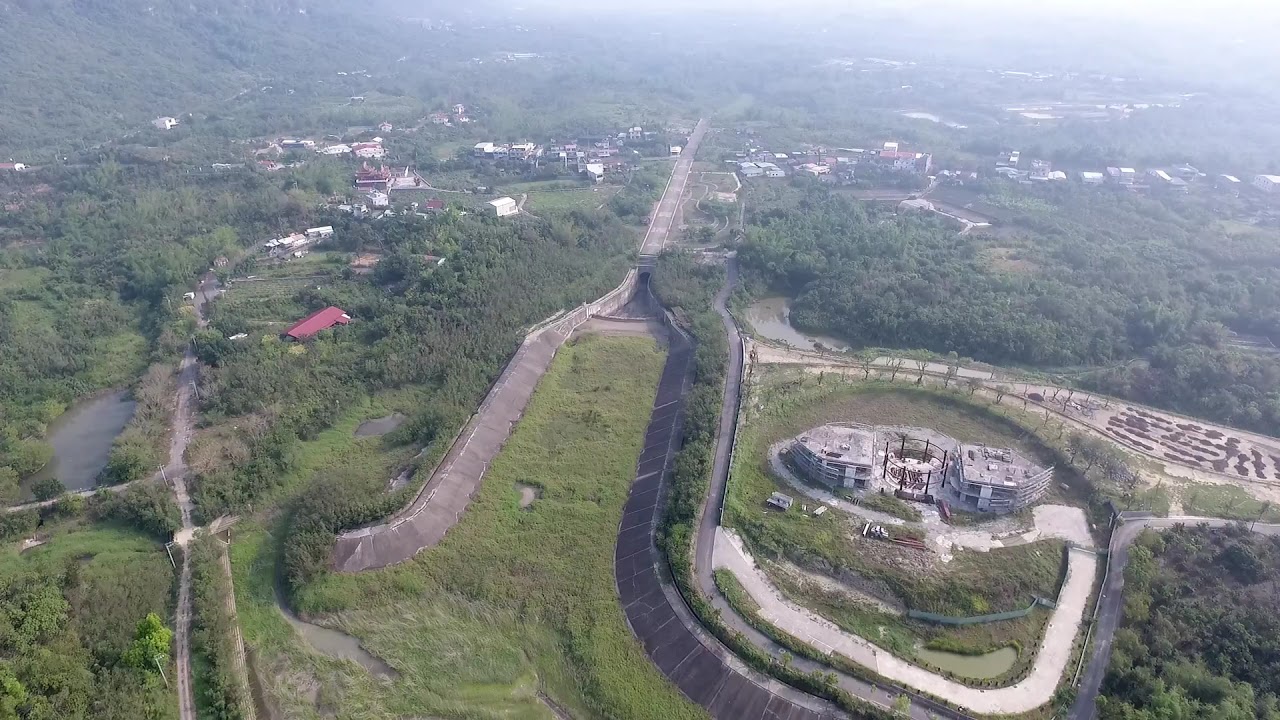This high-definition, wide-format aerial photograph, taken during daylight hours, presents a detailed landscape of a small to medium-sized town characterized by abundant greenery and scattered low-level buildings. The horizon appears hazy, with no distinct sky visible, giving the upper portion of the image a glared effect. On the bottom right, there's a notable circular developed area with a housing structure at its center alongside a couple of adjoining buildings and a concrete driveway that connects to a main, remarkably straight road, which runs from the bottom left corner to the top center of the image, somewhat resembling a runway. This road is flanked by small houses on either side, leading towards the distant horizon where the image fades into a misty blur. To the left of this central roadway, there's a small body of water, and beyond that, mountains appear faintly at the very edge of the photograph, their exact number indiscernible due to the photograph's framing. The colors in the image span various shades of green, brown, gray, with occasional patches of white, black, red, maroon, and orange, enhancing the natural and structural elements. The bottom right also features a commercial facility, possibly a power plant, distanced from the housing areas. The overall composition, rendered in a realistic, representational photographic style, conveys a serene yet structured snapshot of a town nestled amidst verdant surroundings, captured from a high vantage point.